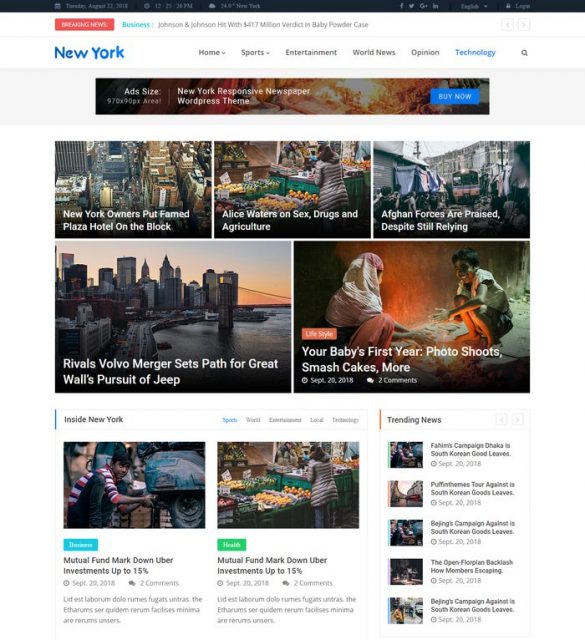An informative and comprehensive caption for the described image would be:

"This image captures a detailed view of a New York-based news website homepage. Dominating the left side is a prominent 'Breaking News' button in red with white text, followed by a green 'Business' section headline announcing 'Johnson & Johnson hit with $417 million verdict in baby powder case.' The top-left corner features 'New York' in bold blue font. The navigation bar to the right includes several sections: 'Home' and 'Sports' both with drop-down menus, along with 'Entertainment,' 'World News,' 'Opinion,' and a highlighted 'Technology' in blue. A search icon is also present, facilitating easy content discovery. Below the headline, there is an advertisement block that reads 'Ad Size, New York Responsive Newspaper, WordPress Theme - Buy Now,' aimed at individuals interested in creating their own newspaper website. The layout includes a gallery of five images, three on top and two below, arranged to form a rectangle. Headlines for these images include 'New York owners put Famed Plaza Hotel on the block,' 'Palace Waters on sex, drugs, and agriculture,' and 'Afghan forces are praised despite still relying,' alongside others like 'Revival's Volvo merger set a path for Great Wall's pursuit of Jeep,' and 'Your baby's first-year photo shoots, smash cakes, and more.'"